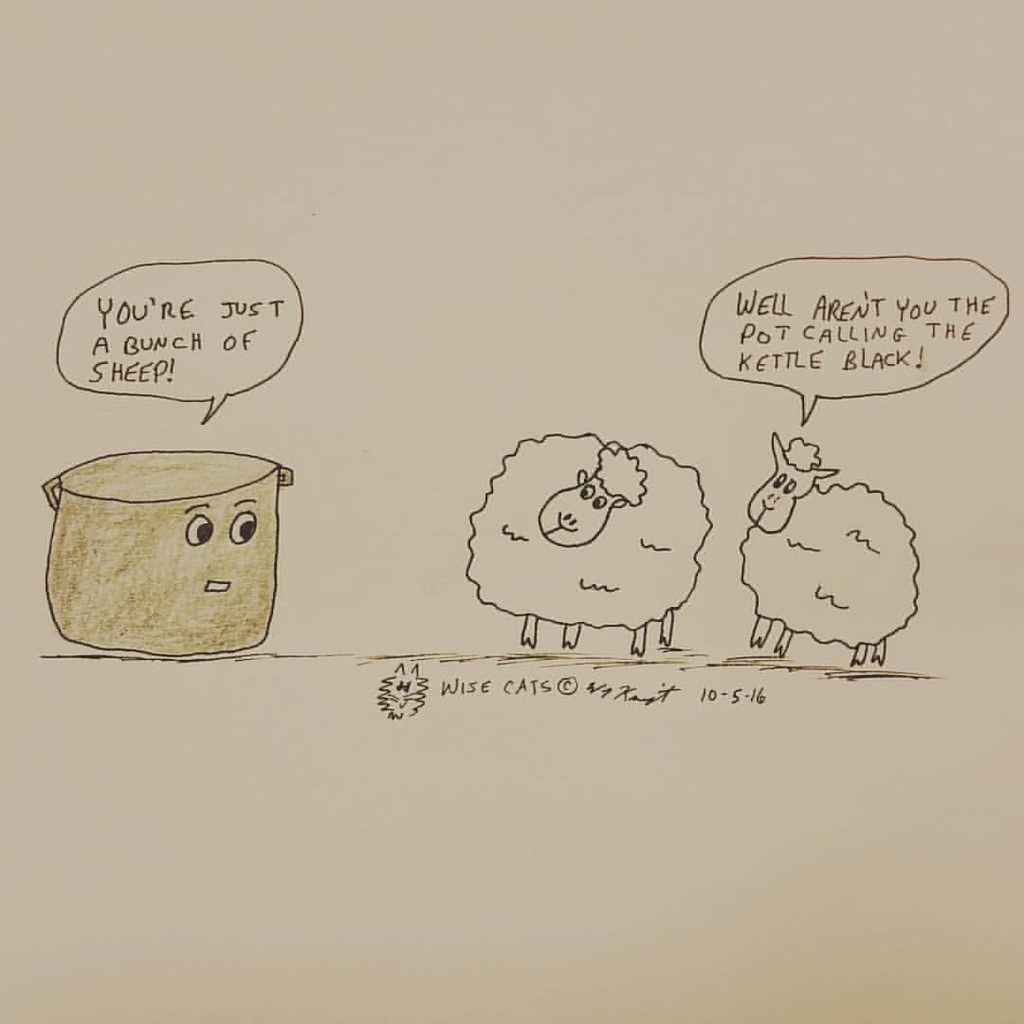This hand-drawn comic, made entirely with pencil and crayon on white paper, humorously depicts a dialogue between a brown pot and two sheep. On the left, the brown pot features eyes and a mouth, and a speech bubble above it exclaims, "you're just a bunch of sheep." The two crudely-drawn sheep, characterized by their big woolly fur and smiles, are positioned on the right. One sheep, on the far right, responds with its own speech bubble: "well aren't you the pot calling the kettle black?" Below the characters, there's a simplistic suggestion of the ground. The comic is credited at the bottom with the name Wisecatz, a copyright symbol, and the date 10-5-16, along with an artist's signature. The overall style is reminiscent of simple and humorous newspaper comic strips.